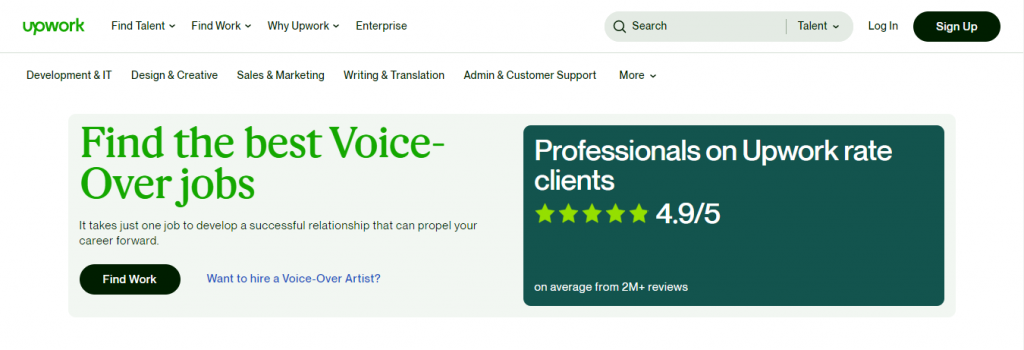The front page of the Upwork website features a clean and organized layout. In the upper left-hand corner, the Upwork logo is prominently displayed in lowercase letters with a green font. To the right of the logo, there are several navigation menus arranged horizontally. The "Find Talent" menu is the first, presented as a drop-down option. This is followed by the "Find Work" drop-down menu and the "Why Upwork" drop-down menu, each providing additional resources and information. The "Enterprise" menu comes next in the sequence.

On the right side of the page, near the top, there is a functional search bar. Within this search bar, there's a drop-down menu labeled "Talent" to refine search queries. Adjacent to the search bar are the "Login" and "Sign Up" buttons, with the "Sign Up" button highlighted in black to attract new users.

Below this top navigation, there's a more detailed menu featuring various categories of services. These categories include "Development and IT," "Design and Creative," "Sales and Marketing," "Writing and Translation," and "Admin and Customer Support." Additionally, there's a visible block that highlights the professional caliber of freelancers on Upwork, stating, "Professionals on Upwork. Great clients, 4.9 out of 5 stars."

This organized and detailed layout helps users navigate the site efficiently, providing clear pathways to the various resources and services offered by Upwork.